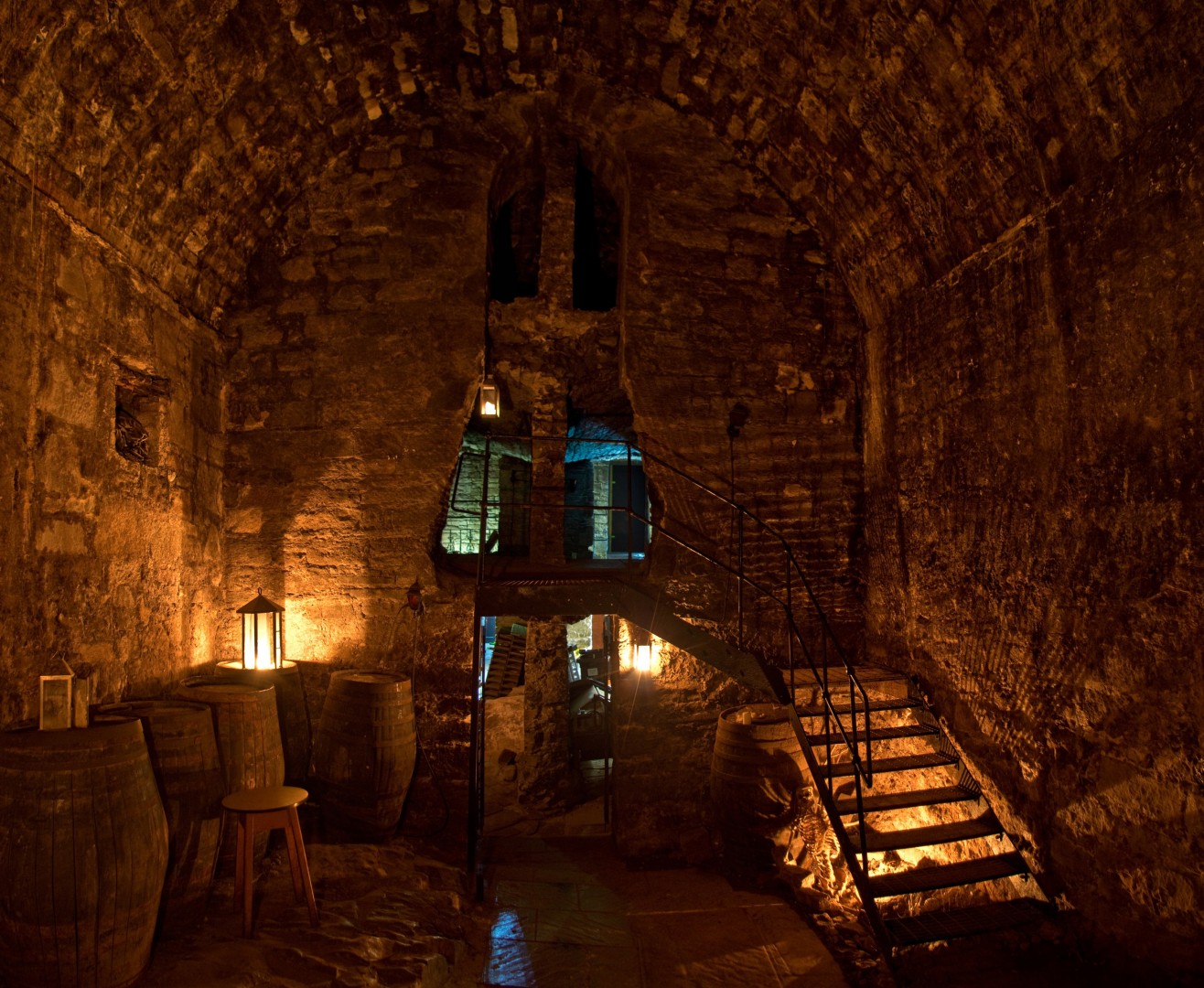The image depicts the interior of a dimly lit, cavernous room, likely within an old stone house or a makeshift structure resembling a temple. The space is predominantly constructed from brownstone with an arched ceiling and features several cutouts at the top, from which lanterns with yellow lights hang, casting a warm glow. The room is characterized by its rugged, ancient appearance, with stone walls and a stone floor adding to the ambiance.

In the lower left corner, there is a small stool adjacent to several tall, cylindrical brown barrels lined up against the stone wall, and a picture frame perched atop these barrels. On the right side of the image, metal stairs ascend from the lower right, curving towards the center and continuing upwards towards the left, leading to another stone level visible in the background.

The colors captured in the photograph include shades of teal, light blue, black, yellow, orange, brown, light brown, and beige. There are openings in the stone wall that suggest pathways to other parts of the structure, contributing to the overall sense of antiquity and mystery. The lighting and the interior setup evoke an inviting, yet enigmatic atmosphere inside this spacious room.